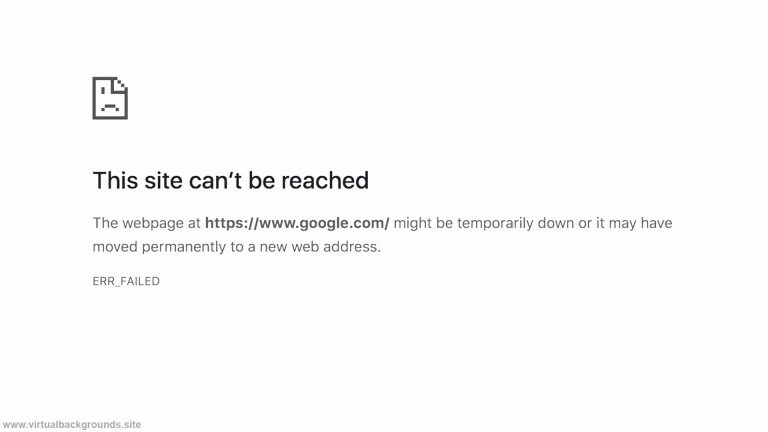The image depicts a frustrating scenario for internet users: a plain error page displayed when a site cannot be accessed. Set against a light gray background, the most prominent feature is a rectangular box with a folded corner, in front of which an unhappy face icon is situated. Dominating the box are large, black, bold letters stating, "This site can't be reached." Directly beneath this, in bold text, it reads, "The webpage at https://www.google.com/ might be temporarily down or it may have moved permanently to a new address." Below this message, an error code is displayed in all caps: "ERR_FAILED."

The page is otherwise stark and unembellished, adding to the user's frustration. In the bottom left corner, in small text, is the URL "www.virtualbackgrounds.site," providing no additional context or information. This barren notification leaves the user with a sense of abandonment, urgently signaling that the site is unreachable without offering a clear resolution.